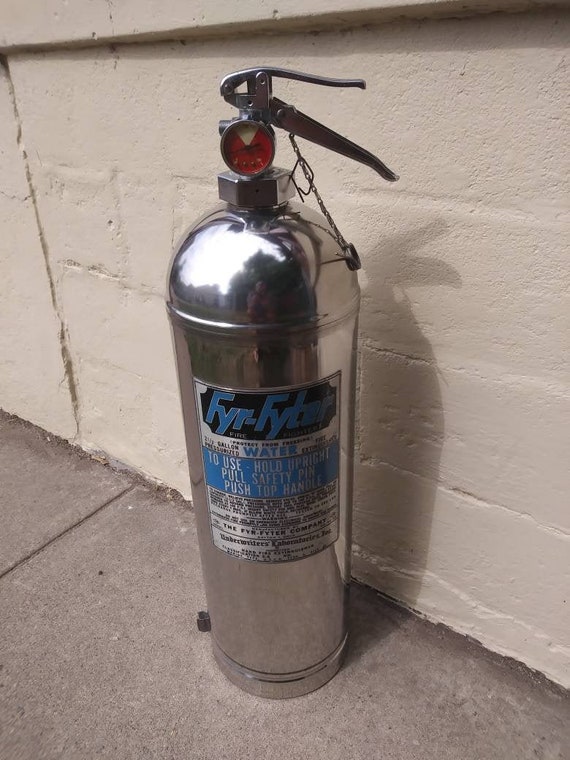This vertically aligned rectangular photograph shows an older, chromed silver fire extinguisher positioned against a painted brick wall. The wall, predominantly white with a slight beige tint, provides a textured background that highlights the shiny metal canister. The fire extinguisher is standing on a gray concrete sidewalk. 

At the top of the fire extinguisher, there is a rounded pressure gauge with a red section and a small white segment, indicating the pressurized contents inside. Attached to the top is a squeeze trigger handle, which features a small circular red shape at the front and a chain hanging down. 

On the cylindrical body of the extinguisher, there is a prominent square label in blue, black, and white colors stating “F-Y-R dash F-Y-T-E-R” in blue block letters against a black background. Below this, the label indicates the contents as water in blue letters and provides usage instructions: "To use, hold upright, pull safety pin, push top handle," printed in gray letters against a blue background. The detailed labeling and unique chrome finish set this fire extinguisher apart from the more common red ones, providing a functional and aesthetically interesting focal point in the image.